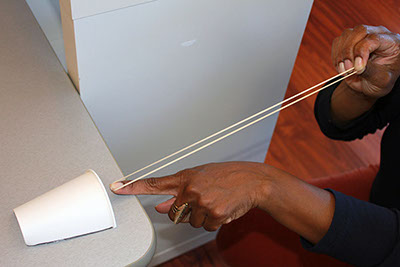The photograph captures a detailed, mid-action moment of a dark-skinned man sitting in a room with a rich brown-red hardwood floor and pulling back a stretched, light brown rubber band. He is wearing a navy blue shirt and red pants. His hands, one of which bears a ring, display signs of age as he aims the rubber band at a white paper cup positioned near the edge of a gray, plastic-looking counter. The counter is set against a white wall, and the man's left hand helps steady the rubber band while his right hand pulls it back, ready to release. The overall scene is intimate, with the focus on the taut rubber band, the simple white cup, and the concentrated effort of the man's hands. The gray counter and hardwood floor contrast with the vividness of his attire, making the whole scene pop.